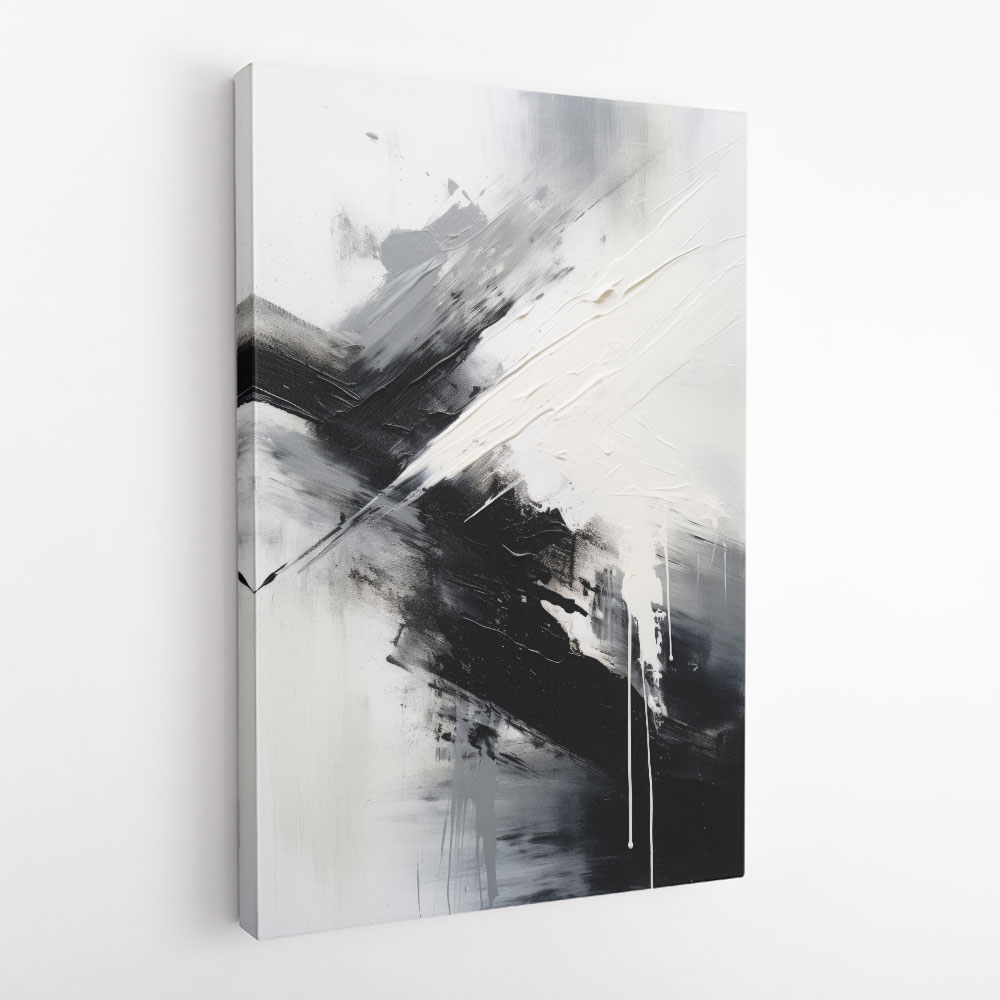This image shows an abstract painting hanging on a white wall. The painting is an unframed canvas, predominantly featuring a backdrop of blended white, gray, and black paints. The composition appears chaotic, with splashes, streaks, and dots of varying shades. White paint drips down from the top, evocative of snow or mist, while the black and gray areas create a textured, mountainous impression. Though this abstract piece does not follow any specific form, the interplay of colors and patterns suggests a dynamic, almost natural scene, possibly resembling a mist-covered mountain during the day. The dried paint textures further enhance the complexity and depth of the artwork, making it a striking visual element against the plain white wall.